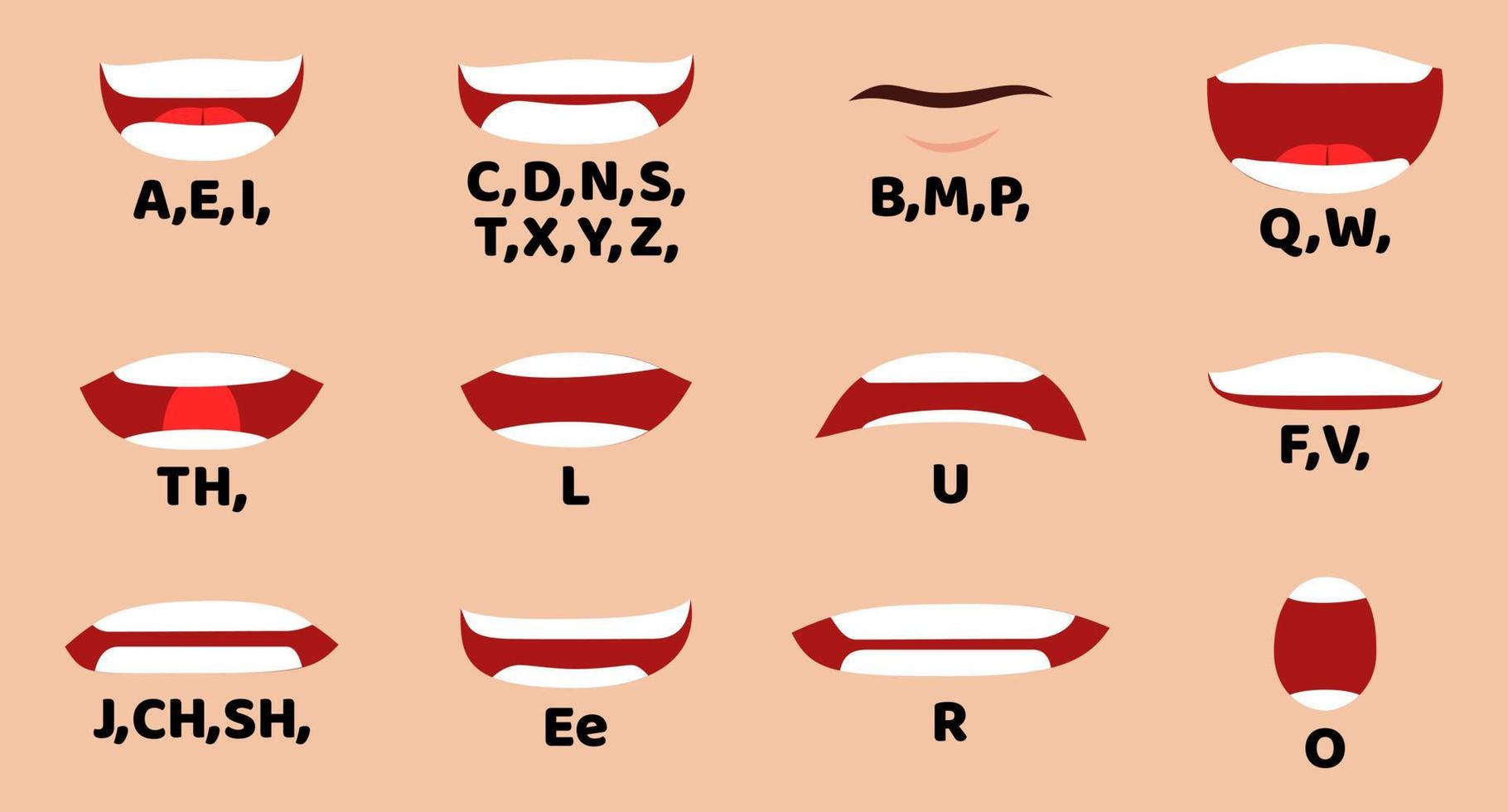This detailed illustrated diagram features 12 configurations of a mouth against a pale orange background, each labeled with distinct letters in black text. The first image shows a slightly open mouth revealing a bit of tongue and white teeth, labeled AEI. To the right, a mostly closed mouth displays no tongue but visible teeth, labeled CDNSTXYZ. Following that is a closed mouth with just a brown lip, labeled BMP. Next, a very wide open mouth showing both tongue and teeth is labeled QW.

In the center row, starting from the left, there is an open mouth with teeth visible and the tongue spanning vertically, labeled TH. To its right, an open mouth with teeth visible but no tongue, labeled L. This is followed by a frowning mouth with visible teeth, labeled U, and then a smiling mouth showing only the top row of teeth, labeled FV.

The bottom row begins on the left with a wide open mouth showing only teeth, labeled JCHSH. To the right of this, a smiling open mouth without a visible tongue, labeled EE. Further right is another wide open mouth showing only teeth, labeled R, and finally, a very tall open mouth without a visible tongue, labeled O.

These mouth shapes and their corresponding labels suggest a phonics-related illustration, focusing on the articulation of different sounds.